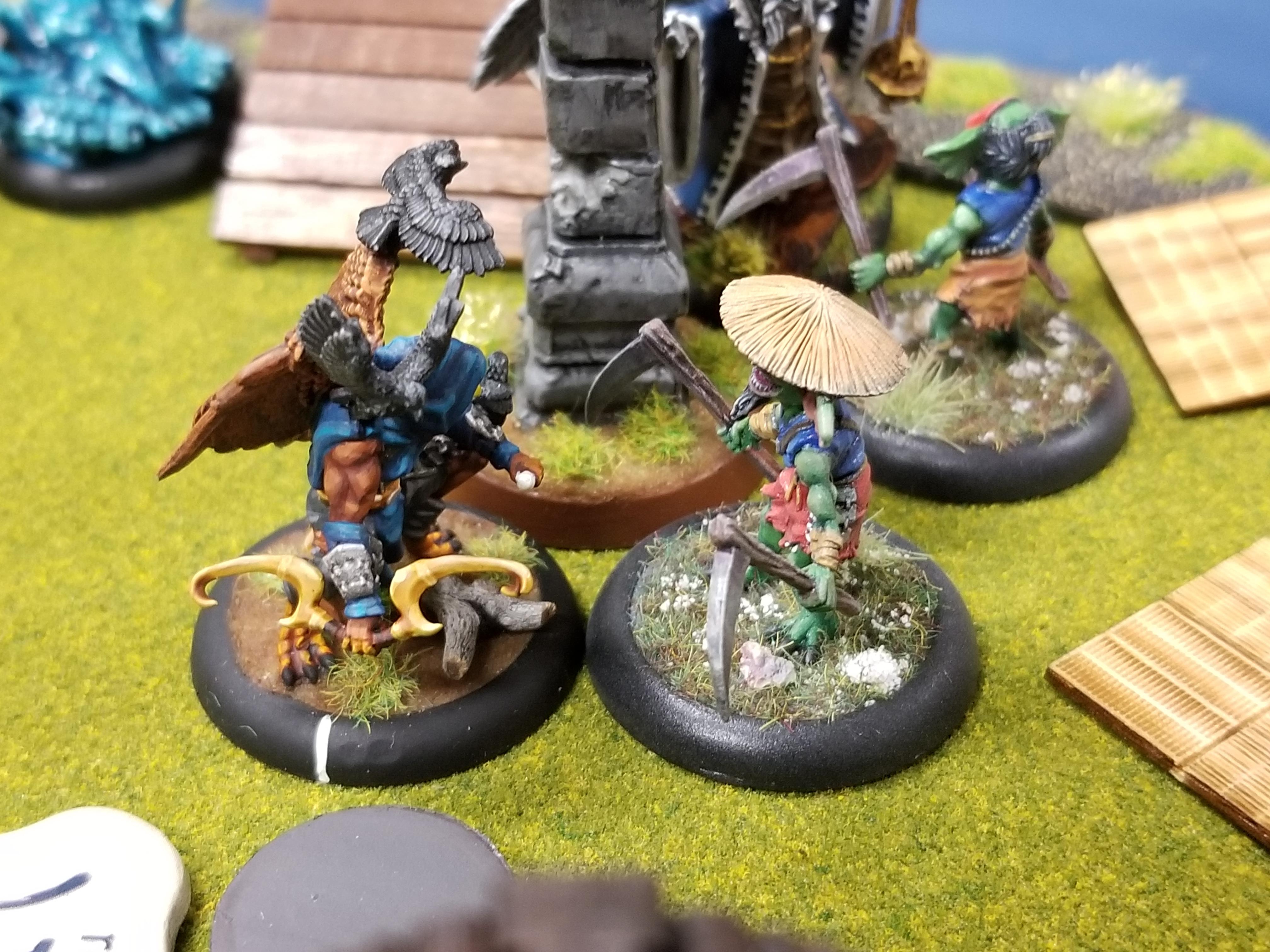The color photograph depicts a collection of intricate figurines arranged on a green, grassy-like surface, possibly resembling a placemat or table cover. The figurines, which appear to be either cartoonish or animated characters turned into silver-plated or silver-painted sculptures, are mounted on round black platforms with grassy bases.

In the middle, a prominent figure stands holding two sickles, dressed in a blue top and red pants. To the left, another figurine features gray birds perched on its shoulders and brown wings, also wearing a blue top and holding a yellow object. Behind these, on the left, there is a figure with some monstrous features, clad in a blue cloak. To the rear right, another figurine with semi-human features has green arms, a black top, and a brown garment, possibly wielding a weapon. Additionally, there are brown wooden squares, perhaps crates, scattered in the background.

The overall scene is set against a blue backdrop that appears almost watery, contributing to a mystical ambiance. The meticulous detailing, from the gray birds and brown wings to the green arms and blue capes, underscores the craftsmanship of these collector’s items.